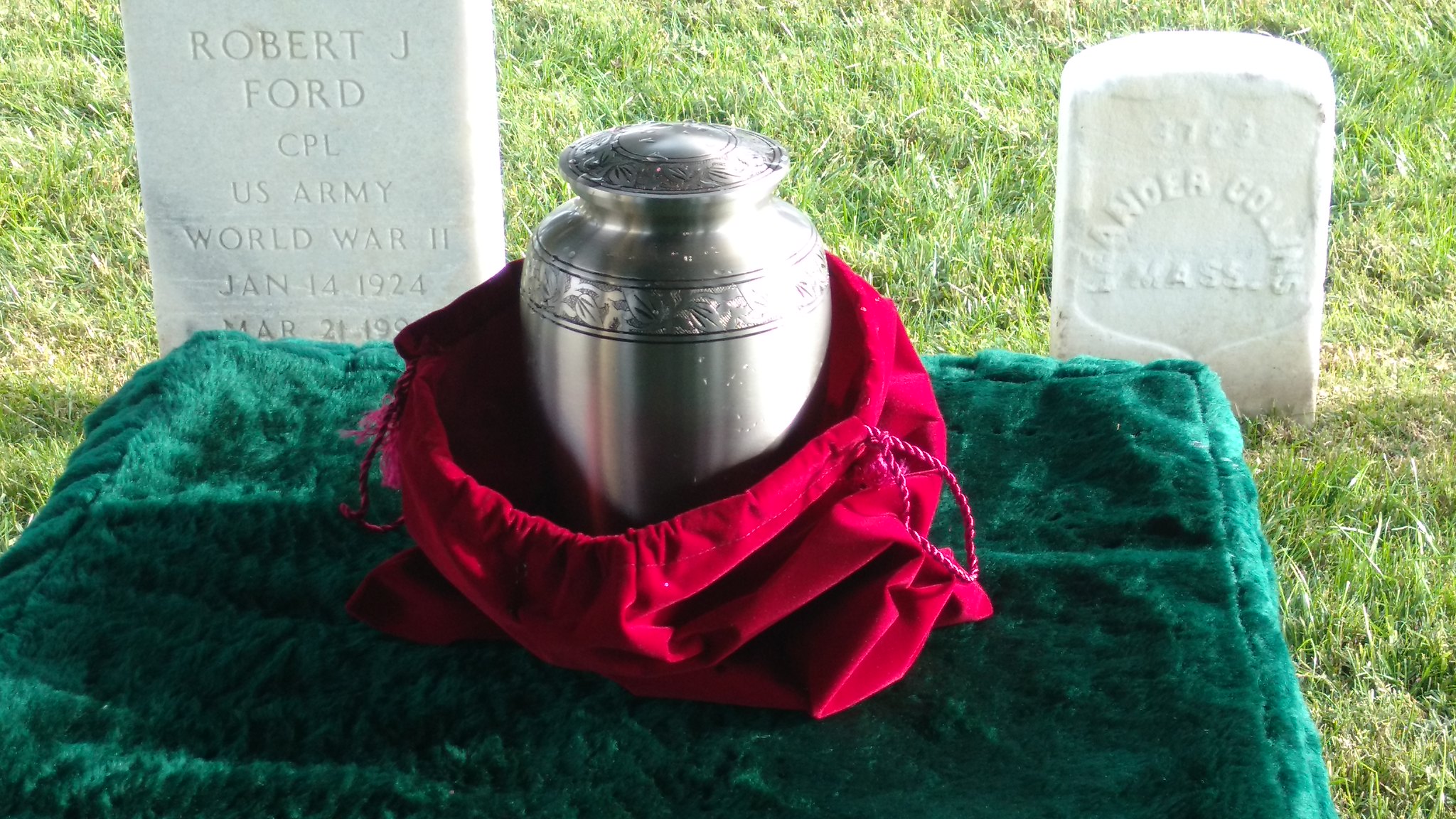In the photograph, there is a serene cemetery scene featuring two gravestones under a bright, sunny sky. The gravestone on the left is taller and engraved with the details: "Robert J. Ford, CPL, U.S. Army, World War II, January 14, 1924 - March 21, 1990." The gravestone on the right is shorter and more worn, making it difficult to discern the complete inscription, though it appears to read "Hander Collins", possibly another war veteran. In front of these gravestones lies a green fur mat with a silver urn placed atop it. The urn, potentially holding the remains of the deceased, is partially covered by a red velvet-like bag resembling a satin Ziploc sack. The scene is tranquil, highlighted by bright sunlight illuminating the green grass, adding a gentle, reverent atmosphere to the image.